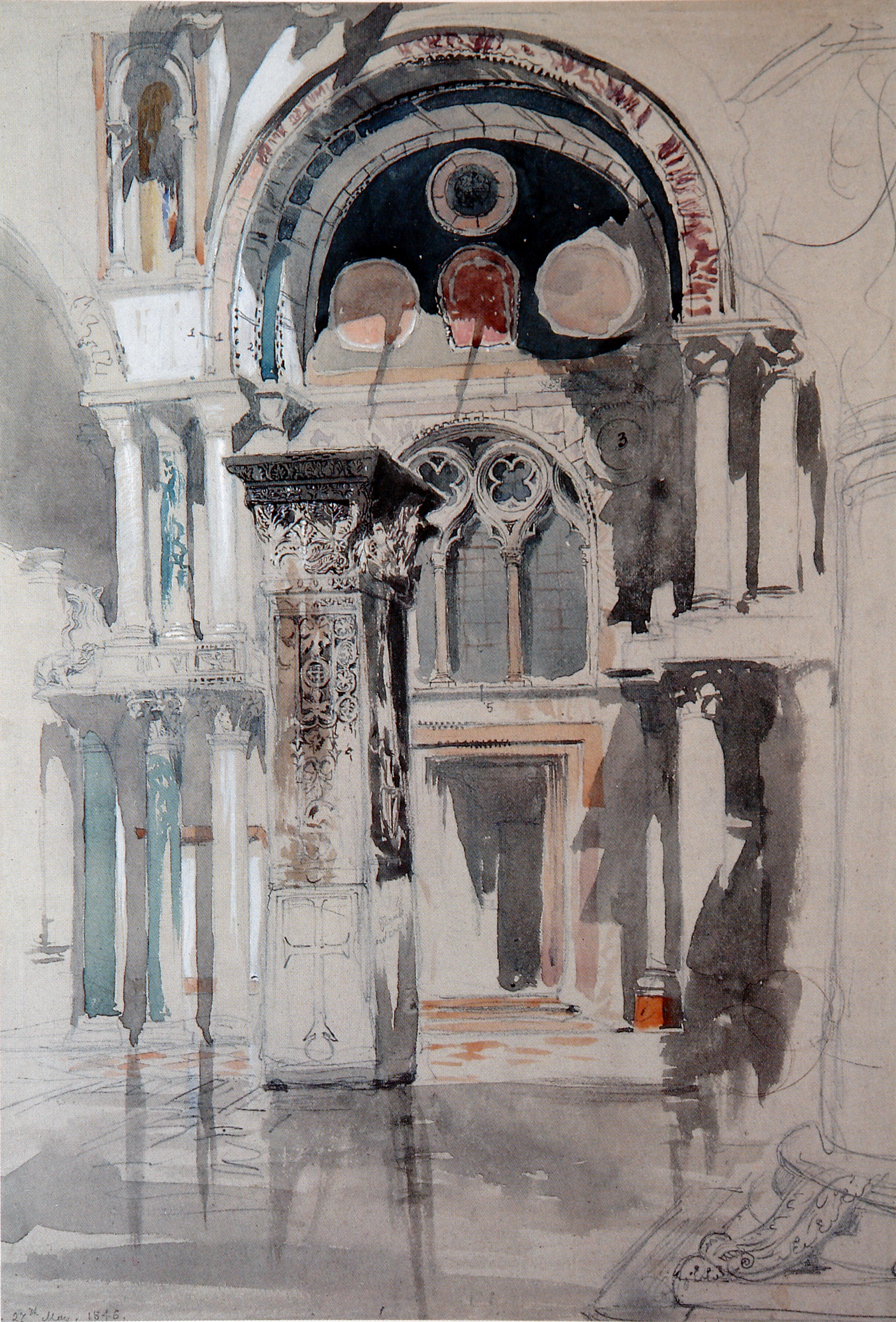The image depicts what seems to be the stately exterior of a church, captured in a washed-out palette of bright, muted hues. Central to the scene is a large Promethean arch adorned with circular windows and columns at its peak, suggesting an intricate facade. The middle section features a grand church window with stained glass, adding a splash of vibrant reds and greens amidst primarily neutral tones. Below the window stands a large ornate door, flanked by a series of columns that frame the entrance. In front of the door is a notable post, adorned with a cross and detailed carvings. The scene, enclosed within a rectangular frame, presents an amalgamation of refined architectural details reminiscent of Renaissance Italy, with a courtyard-like tiled floor that reflects light, hinting at a polished surface. Although the exact location within the church—inside or out—remains ambiguous, the grandeur and ornate carvings convey a rich historical elegance.